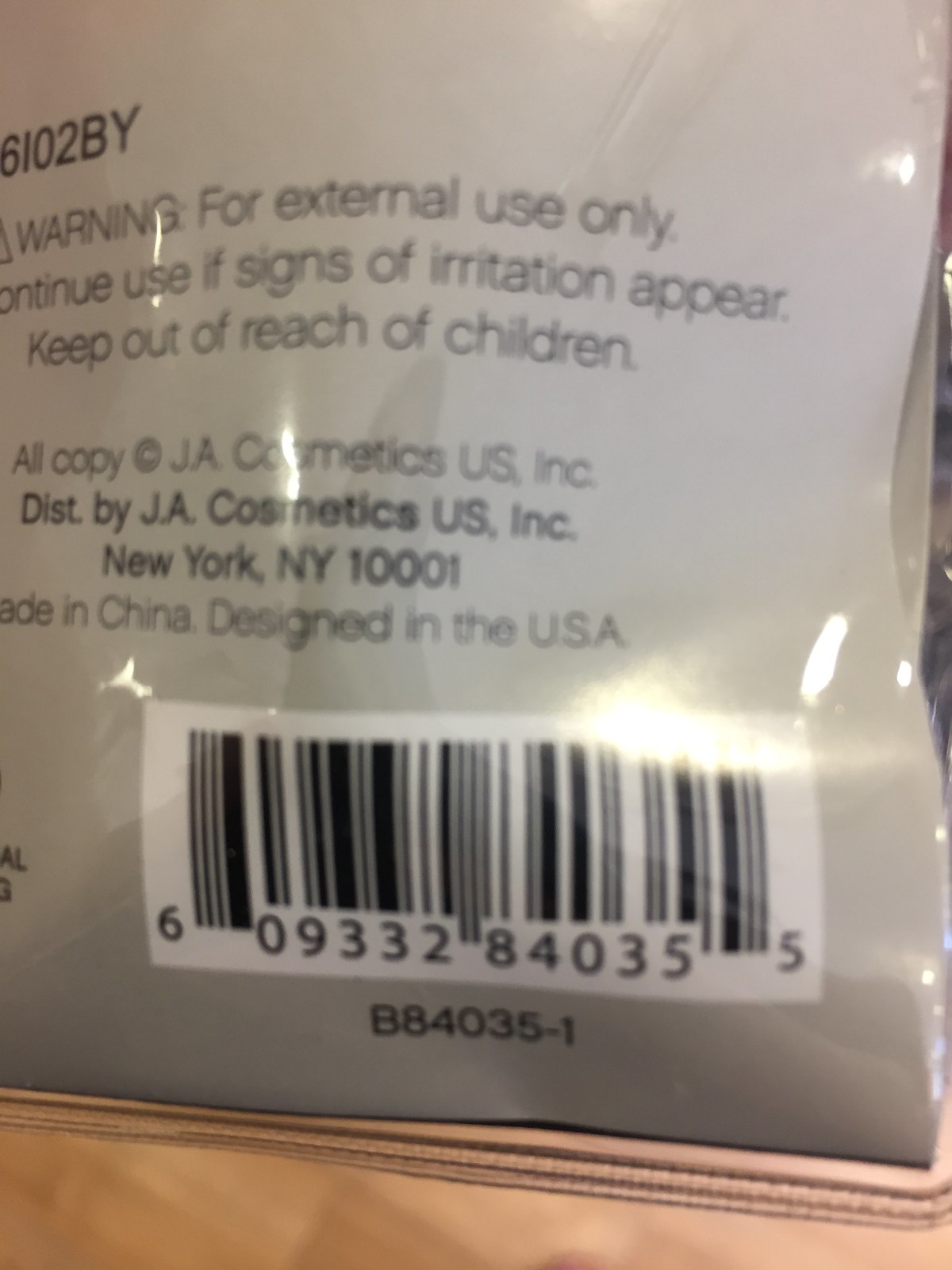This image is a close-up of the back bottom right corner of a product's packaging, made of plastic with a reflective, light gray surface that shows aggressive overhead lighting, causing a strong flashback particularly around the barcode. The packaging is square-like and prominently features a black and white barcode that reads "6 09332 84035 5." Additionally, the background’s white area contains the code "6102BY" at the top left. Printed in black font, the text includes safety and manufacturing details: "Warning for external use only. Discontinue use if signs of irritation appear. Keep out of reach of children. All copy J.A. Cosmetics US Inc. Distributed by J.A. Cosmetics US Inc. New York, New York 10001. Made in China. Designed in the USA." The bottom part of the image shows the package resting upon a very soft, light brown surface.